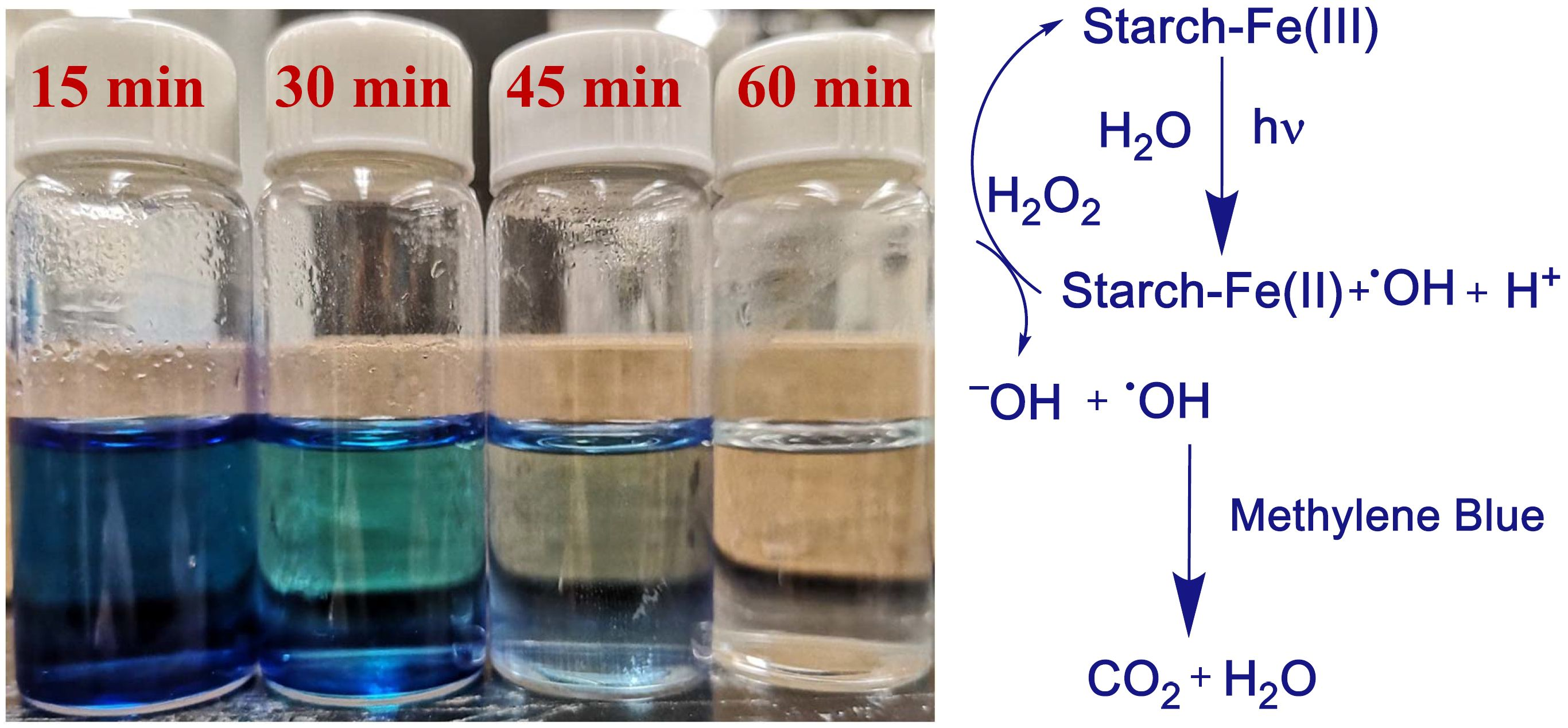The image is a detailed representation of a chemistry experiment. On the left are four clear vials, each filled halfway with a liquid and capped with white lids labeled with time amounts in red: 15 minutes, 30 minutes, 45 minutes, and 60 minutes. The liquid colors transition from dark blue in the 15-minute vial to lighter blue at 30 minutes, very pale blue at 45 minutes, and clear at 60 minutes. On the right side of the image is a chemical diagram with text in blue, detailing a reaction involving starch, methylene blue, CO2, and H2O. The diagram shows a progression from starch (Fe) to methylene blue, indicating the transformation process over time. The layout provides a visual comparison between the color changes in the vials and the corresponding chemical reactions described in the diagram.